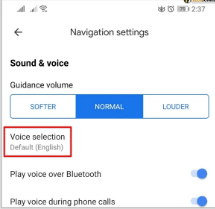This image is a low-resolution screenshot taken from a mobile phone, featuring a white background. At the top, various gray icons provide current phone information: on the right, there is an alarm clock icon, a battery icon displaying '75%', and the time indicated as '2:37'. On the left, Wi-Fi and mobile data icons are fully illuminated. Below these icons, in black font, the text "Navigation Settings" appears, accompanied by a left-pointing black arrow.

Beneath this header, a bold black text reads "Sound and Voice", followed by "Guidance Volume" in regular black font. Here, a blue-outlined rectangle is present, containing blue text with options "Louder", "Normal", and "Softer". The "Normal" option is selected, highlighted by blue outlining.

Further down, a red box surrounds the text "Voice Selection", with "Voice Selection" in black font and "Default English" in gray font. Underneath, the options "Play voice over Bluetooth" and "Play voice over phone calls" are listed, both of which have been selected.